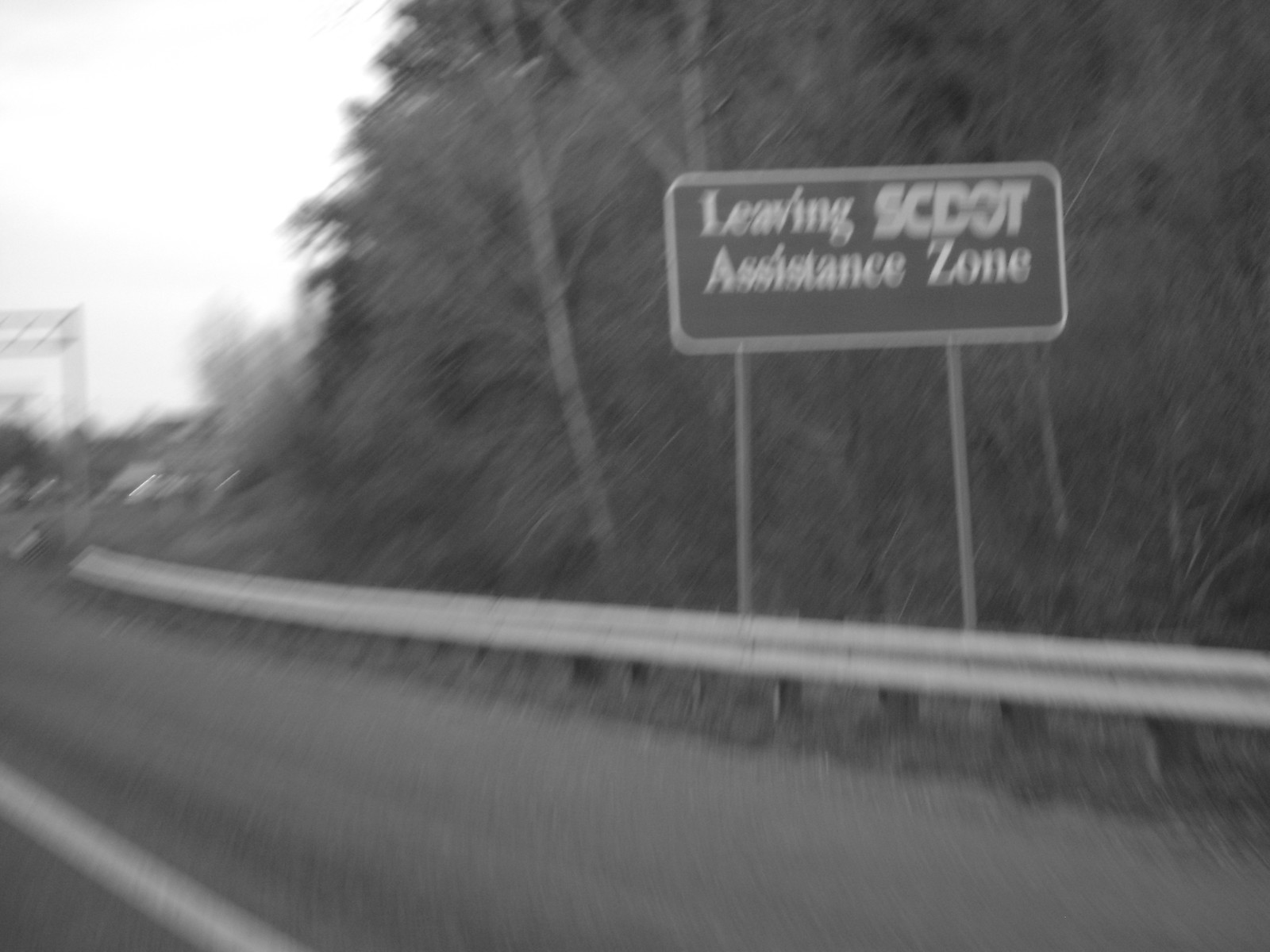This blurry black and white photograph captures a roadside scene from a vehicle traveling along a highway. A long metal guardrail runs horizontally across the image, preventing vehicles from veering off into the heavily wooded area in the background. The dense foliage is primarily composed of tall trees and thick leaves, with only a few tree trunks visible through the greenery. Dominating the scene is a large rectangular street sign supported by three legs that reads, "Leaving SCDOT Assistance Zone" in white text. Near the bottom left corner of the photo, part of a white line can be seen diagonally marking the edge of the road. Additionally, there appears to be another metal structure or sign partially visible further ahead. The sky in the top left corner is white, adding to the overall monochromatic and slightly unfocused appearance of the image.